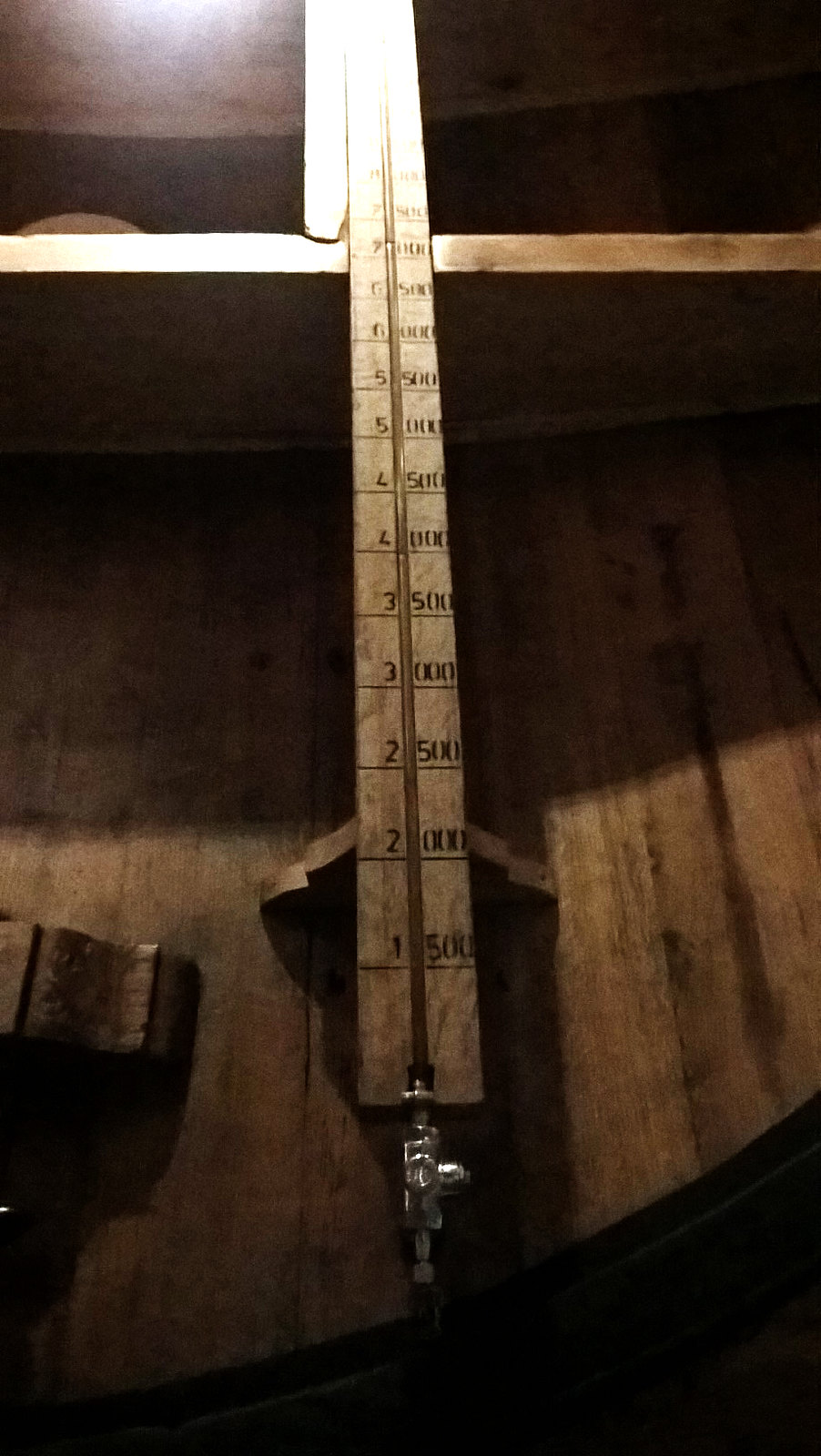The image depicts a detailed setup of a scale situated on a round wooden table, which is evident from the curvature observed at the bottom edge of the image. The table supports various components of the scale. Central to the image is a vertically oriented ruler, mounted on small wooden supports. At the base of the ruler, there seems to be a metallic component resembling a spout.

The ruler features multiple numerical markings: on the left side, sequential numbers from 1 through 7 are visible, increasing by increments of one. The markings on the right side, however, alternate between 500 and 0, progressing in increments of 500 from 500 to higher values such as 1500, 2000, 2500, continuing up to 7000. A small light reflection obscures some additional details at the top of the ruler.

Additionally, there is a divot in the middle section of the ruler. At the height marked by 7000, a shelf extends beneath the ruler, supported by an extra piece of wood to the left. This shelf is significantly thicker compared to the bottom supports of the ruler. The intricate assembly and precise markings suggest a scale used for detailed measurements or balancing tasks.